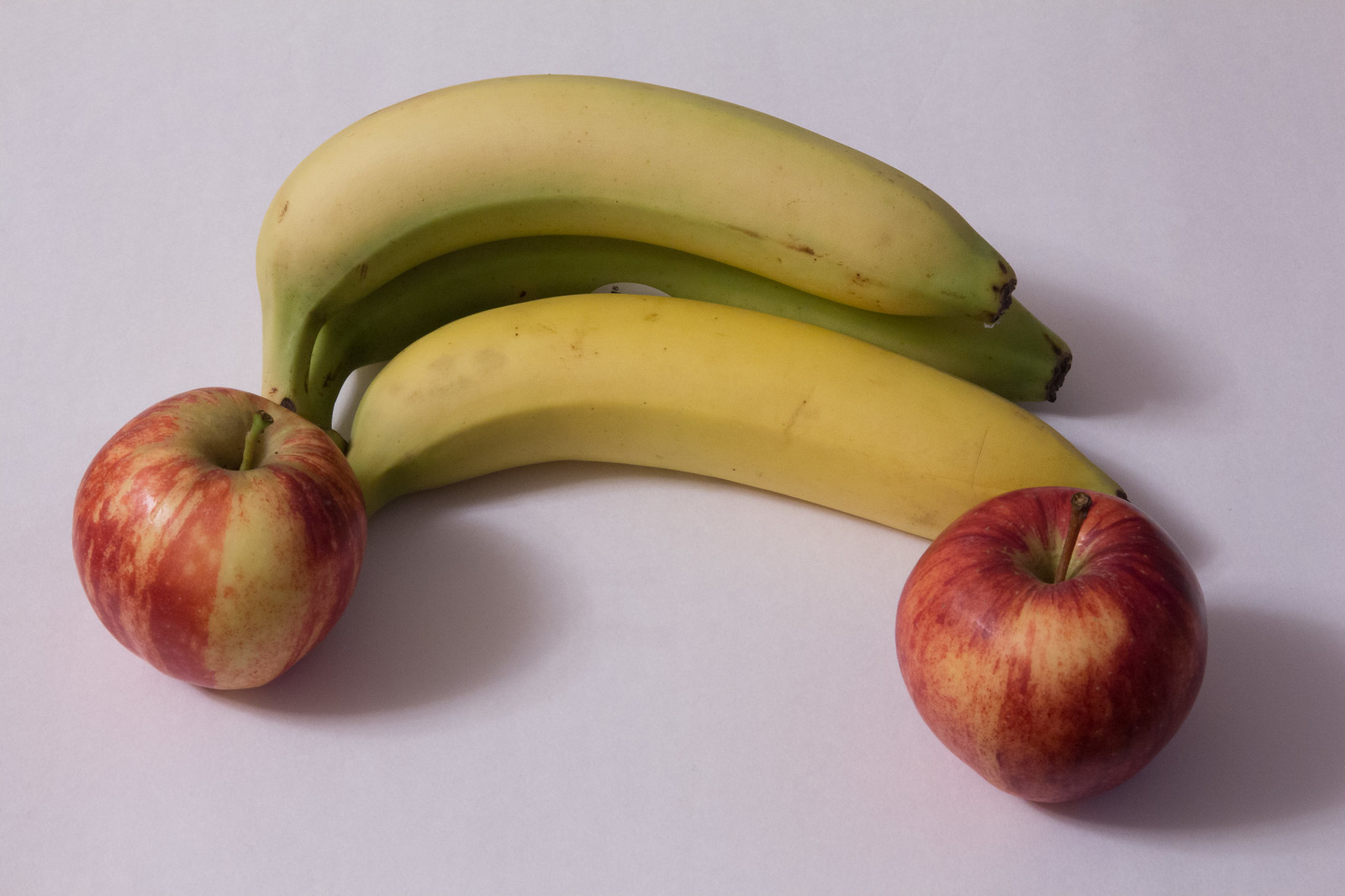The photograph showcases a simple fruit arrangement featuring two apples and three bananas still attached to a larger stem. On the left-hand side of the image stands a single apple, mirrored by another apple positioned on the right-hand side. Centrally placed between the two apples is the cluster of bananas. Among these, the bottom banana is partially obscured, revealing a greenish tint. Above and slightly to the side of it, lies another banana with a faint green line transitioning into a predominantly yellow hue, its tip adorned with small brown spots. The third banana, also mostly yellow with subtle streaks of very light brown, is positioned on its side, arching gracefully to create a visual connection between the two apples. This careful arrangement highlights both the contrast and harmony between the different fruits, with each banana curving naturally to bridge the gap between the upright apples.